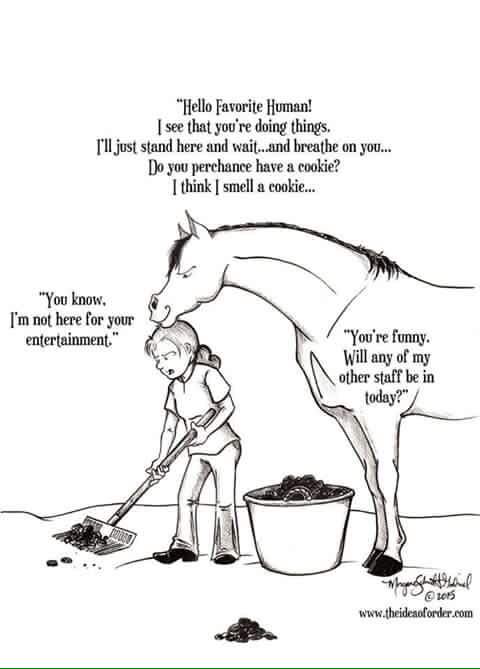In this cartoon-style illustration set against a white background, a young girl is visibly annoyed as she uses a rake to shovel piles of horse manure into a large bucket. Around her, scattered mounds of manure emphasize the unpleasantness of her task. Behind her stands a horse with a menacing grin, watching her intently. Above the horse's head, text reads, "Hello, favorite human. I see that you're doing things. I'll just stand here and wait and breathe on you. Do you perchance have a cookie? I think I smell a cookie." The horse also has text over its body that reads, "You're funny. Will any of my other staff be in today?" To the left of the girl, there is a speech bubble stating, "You know I'm not here for your entertainment." The bottom right corner of the illustration features the artist's signature along with the URL "www.theideaoforder.com" and the date "2015."